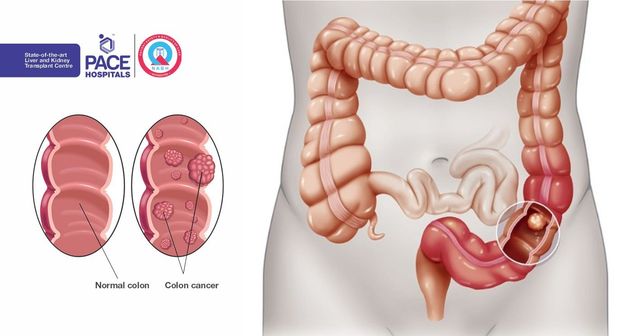The image features a detailed medical diagram depicting a human intestinal tract. On the right side, a grayscale human figure illustrates the position of the intestines, transitioning into a colored diagram highlighting the intestinal tract with beige and red hues. A white circular outline emphasizes an area within the intestines, suggesting the presence of a potential ulcer or cancerous tumor. To the left, the diagram contrasts a "Normal Colon" and "Colon Cancer," where the cancerous colon shows multiple polyps. Accompanying text in blue declares "PACE Hospitals: State-of-the-art Liver and Kidney Transplant Center," with an adjacent red and blue logo.